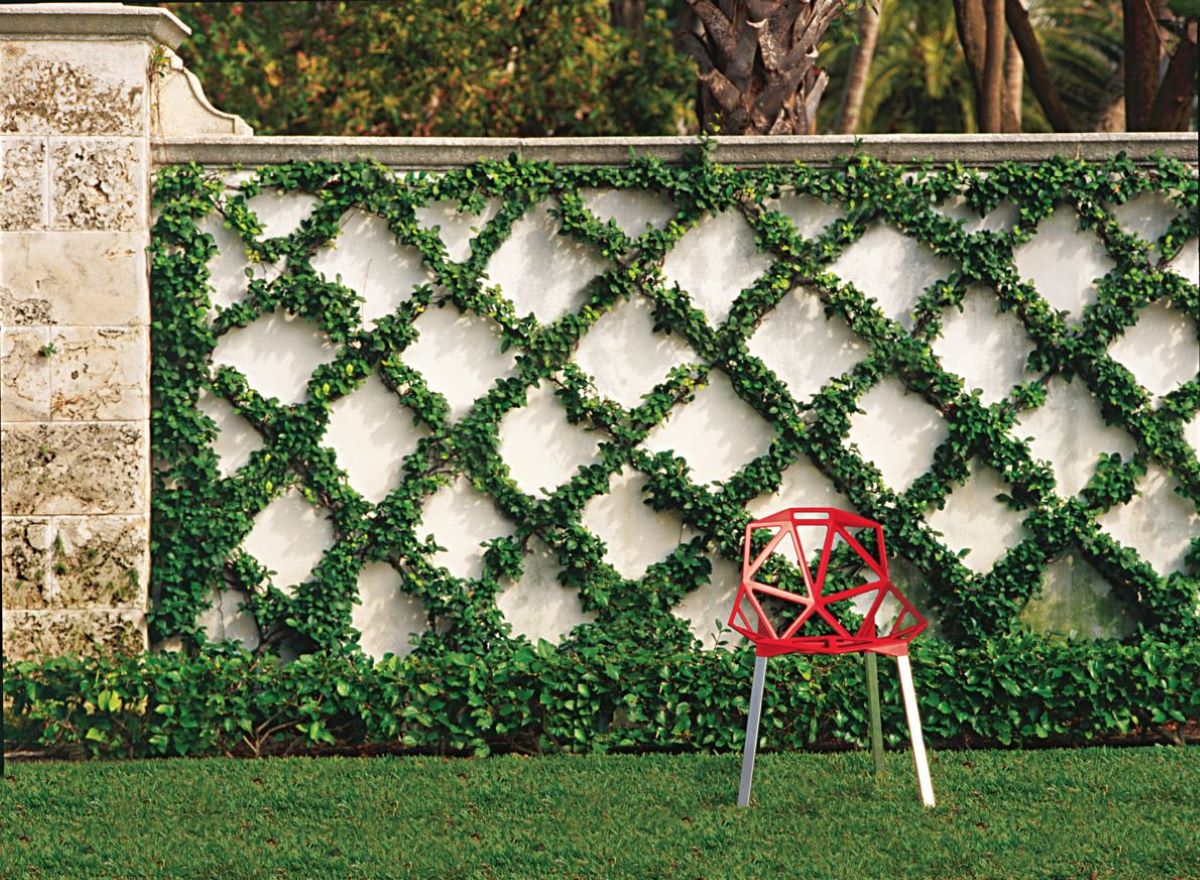The photograph captures the serene backyard of an estate, featuring a large white stone wall adorned with a network of ivy and crisscrossing vines. Central to the image is a high-tech, strikingly designed red chair with an open geometric pattern made up of triangular shapes. The chair features silver metal legs and a distinctive handle-like cutout at the top of its backrest, suggestive of a 3D-printed design. The meticulously manicured grassy lawn stretches across the foreground, and behind the wall, several trees with lush green leaves and brown trunks, including what appear to be palm trees, add to the scene's natural ambiance. The image is brightly lit, likely taken during mid-evening sunlight, highlighting the contrasting textures and colors of the various elements present.